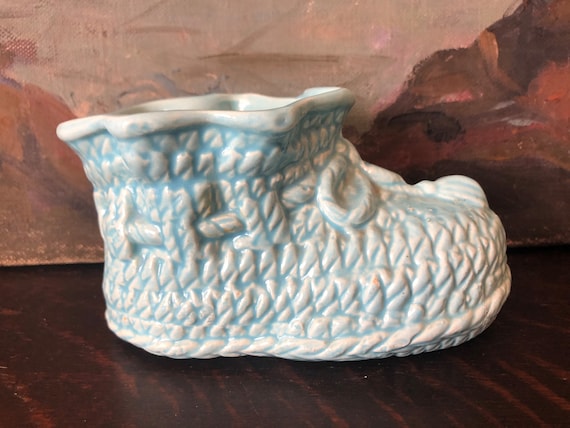The image features a porcelain replica of a baby bootie, designed to mimic the appearance of a knitted shoe. The bootie is primarily white with blue accents, including blue yarn-like patterns and white laces that are tied at the front. The intricate porcelain craftsmanship gives the illusion of a soft knitted fabric, despite being a solid material. The bootie is placed on a sleek, black wooden surface. In the background, there is a painting with a light tan sky and darker brown and black tones, possibly depicting mountains or rocky cliffs. The scene appears to be indoors with no text included in the image.